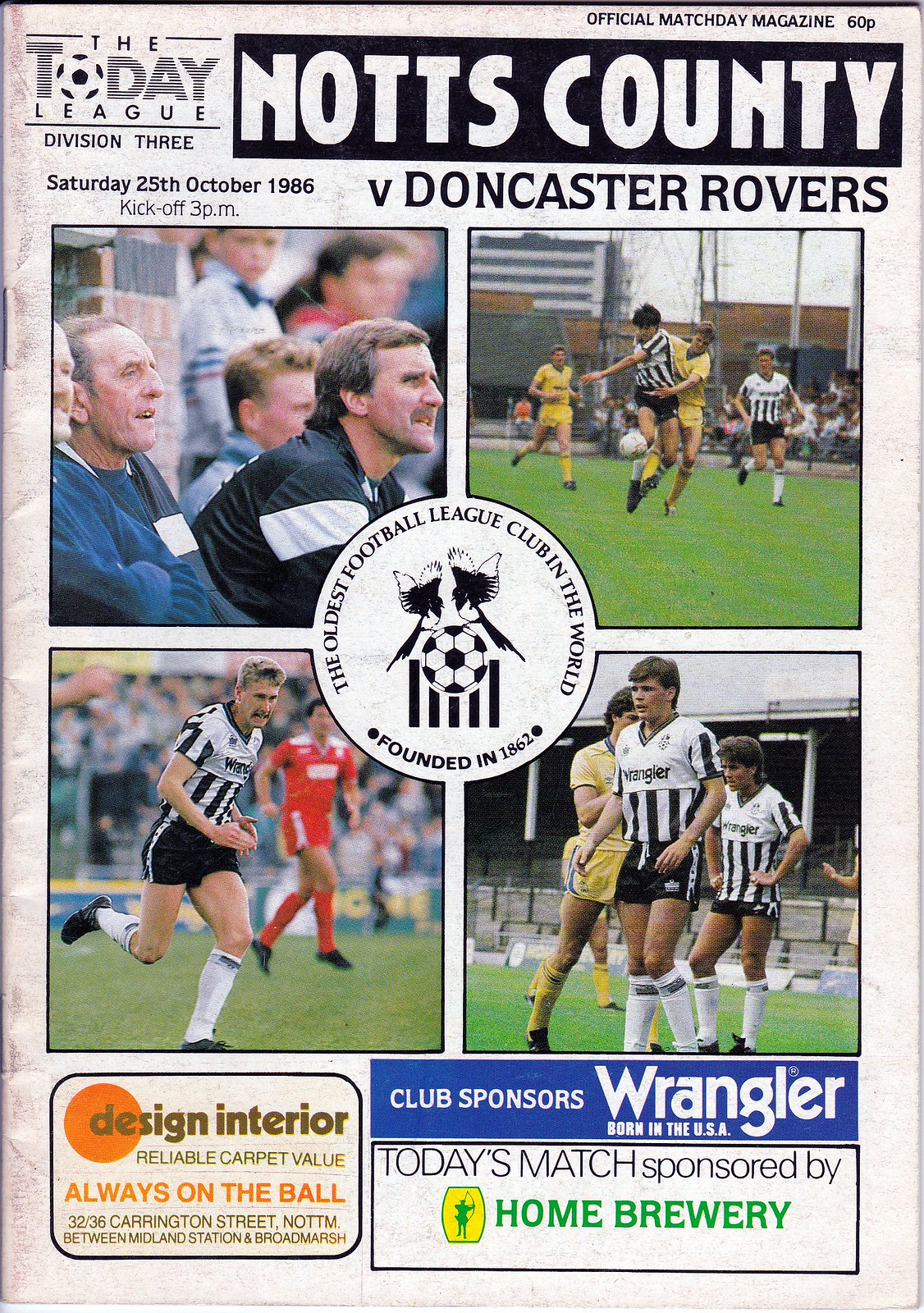The image features the front cover of the official Match Day magazine for the Knotts County football team, titled "Today League." Priced at 60p, the magazine covers the Division III match between Knotts County and Doncaster Rovers held on Saturday, 25th October, 1986, at 3 p.m. The cover is predominantly white and showcases a circular emblem at its center, which reads "The oldest football league club in the world, founded in 1862," decorated with two birds perched atop a soccer ball with five vertical black lines below it.

Surrounding the emblem are four photographs: the top left features the coaching staff, the top right captures a dynamic action shot of a Knotts County player in their iconic black and white vertical striped jersey, facing opponents in yellow. The bottom left image depicts another action scene, with a Knotts County player wearing shorts and white socks, and "Wrangler" emblazoned across his chest. The bottom right image also includes Knotts County players in black and white uniforms, partially shown alongside competitors in yellow and blue.

Below these images, two advertisements are presented. On the left, an orange box promotes "Design Interior - Reliable Carpet Value, Always on the Ball" located at 32-36 Carrington Street, NOTTM, near Midland Station and Broadmarsh. On the right, a blue box with white lettering highlights the club sponsor, Wrangler Jeans, emphasizing "Born in the USA," alongside a note indicating that today's match is sponsored by Home Brewery.